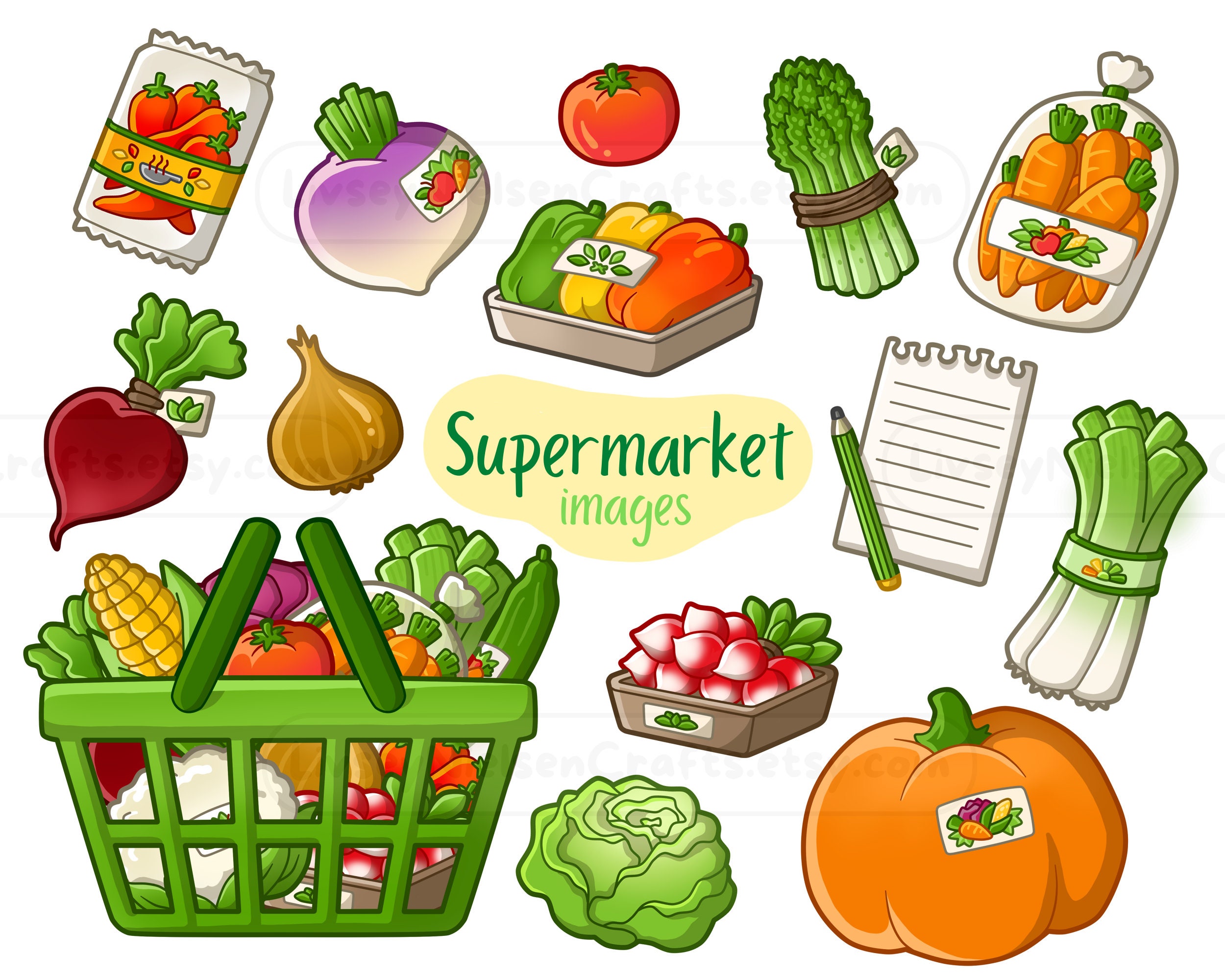This vibrant and detailed cartoon illustration showcases a variety of foods you might find at a supermarket, all set against a white background. In the center, green letters spell out "supermarket" with the word "images" slightly faded and in light green, both encapsulated in an indeterminate yellow blob. Surrounding this central text are numerous colorful vegetable icons. On the left, you'll find radishes, onions, and celery, with a celery bunch and pumpkin further toward the center. Directly beneath the main text, strawberries sit in a metal pan, and a head of lettuce lies below them in the bottom middle. 

In the bottom left corner, a green basket with two handles is filled with an assortment of foods, including corn, tomatoes, carrots, and possibly more celery and radishes. Above the radishes and onion, there’s a package of mixed peppers and another onion, while to the right, a metal pan similar to the one with strawberries contains more peppers, with a tomato just above it. Further right, artichokes are depicted alongside a bag of orange carrots. Below these is a non-food item: a torn-out piece of notepad paper, accompanied by a green pencil without an eraser. 

The illustration features the expected natural colors for each vegetable, along with subtle details like the sticker on the pumpkin and the absence of stickers on the onions. The overall composition and detail suggest a hand-drawn poster, skillfully representing the variety and colorfulness of fresh, supermarket produce.